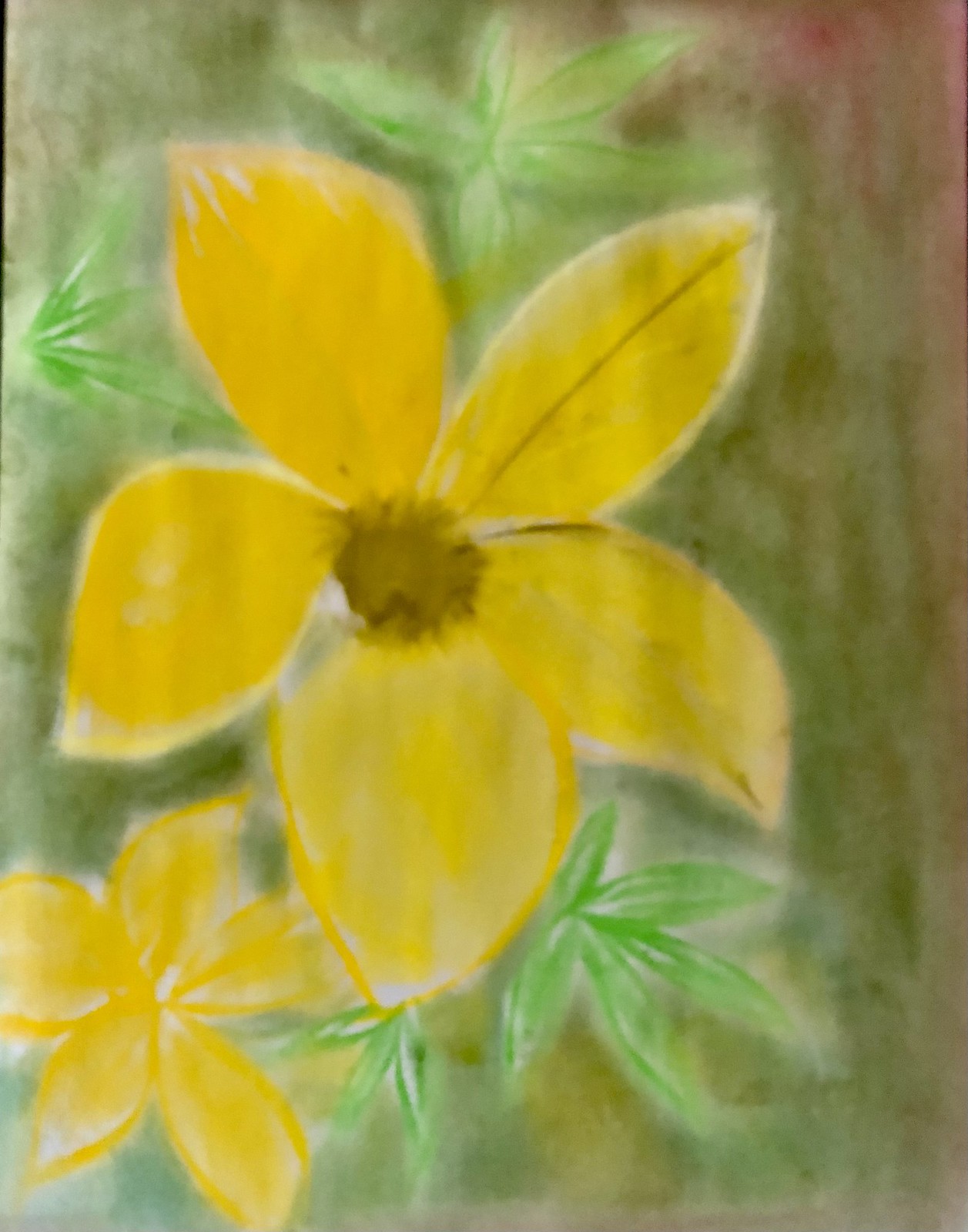This rectangular image, oriented vertically, features a striking painting of a vibrant yellow flower as its focal point. The flower, composed of five bright yellow petals, exhibits a center that blends brown and yellow hues, adding an earthy touch to its vivid coloration. The backdrop is predominantly a deep green shade, interspersed with visible leaves; two positioned at the bottom and two at the top, enhancing the natural ambiance of the scene. Located at the bottom left of the composition, a second yellow flower with equally bright petals appears, significantly smaller in size compared to the primary bloom. Intriguingly, the color palette transitions to a pinkish-red along the right edge of the image, extending upwards and slightly towards the middle, possibly representing a unique tree or another element within the artwork. This contrast in color adds depth and complexity to the overall depiction, drawing the viewer’s eye across the entire canvas.